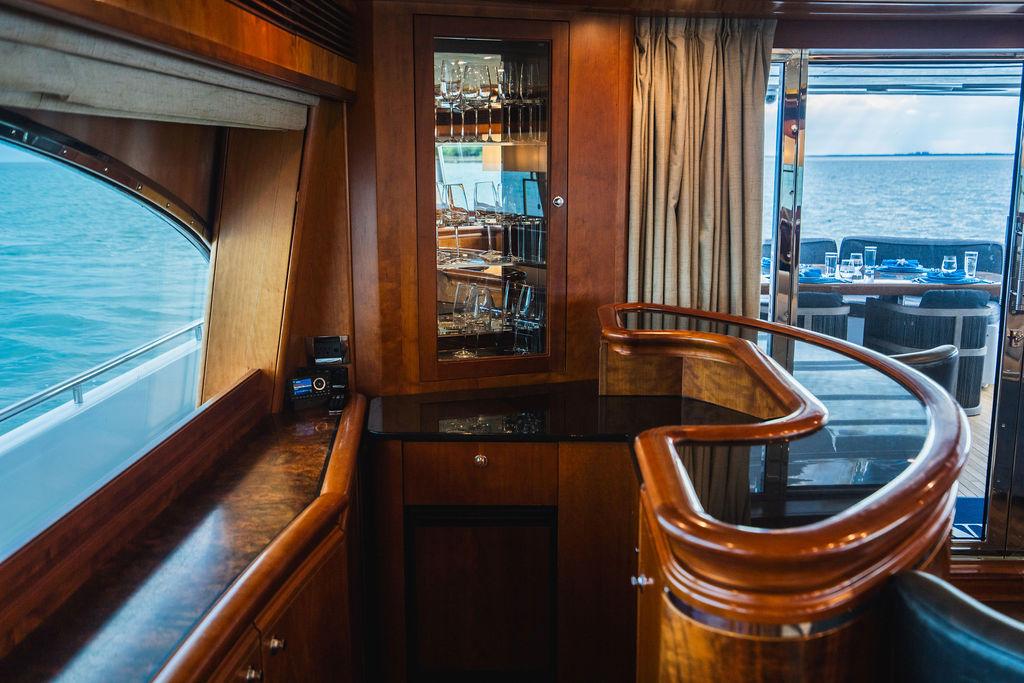The photograph captures the luxurious interior of a large wooden yacht, likely a sailing vessel currently at sea. The scene unfolds with various elegant elements displayed prominently. To the right, a sophisticated wooden bar with a glass countertop stands vacant; no people are visible. Above the bar, there's a cupboard showcasing a collection of wine and champagne glasses, emphasizing the refined atmosphere. Centered in the image, there is a display case holding additional glassware. On the left side of the picture, large windows offer a breathtaking view of the open ocean. There's also a partial view of the boat's exterior deck, furnished with tables and chairs, inviting guests to relax and enjoy the sea breeze. Wooden paneling and fine finishes dominate the decor, underscoring the yacht's opulence. Through the windows, one can spot calm waters and a hint of land on the far horizon, enhancing the serene setting. This image encapsulates the essence of opulent maritime leisure, typifying yacht life.